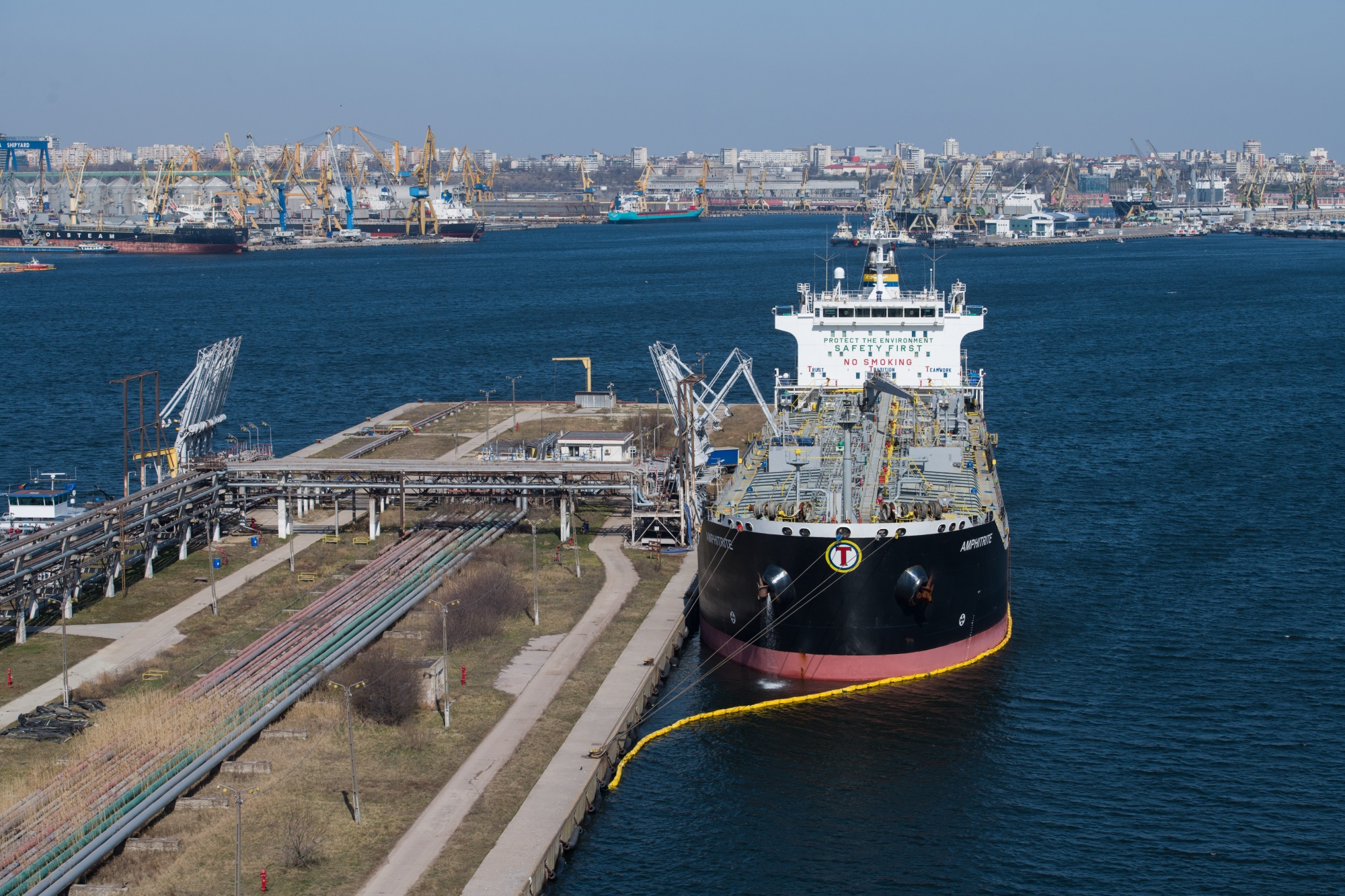The photograph depicts an oil tanker, a large black ocean-going vessel, docked at a port, likely situated along the Black Sea, potentially in Ukraine, Romania, or Moldova. The tanker, with a distinctive red line along its bottom edge, is securely moored to a plain dock equipped with numerous pipes and distribution mechanisms associated with gas or petroleum loading. An orange floating boom encircles the ship to prevent oil spills, indicating active loading or unloading operations. Industrial cranes are visible, assisting in the cargo transfer process, while safety messages such as "Protect the Environment," "Safety First," and "No Smoking" are highlighted on the ship. The scene, captured from an elevated perspective, reveals a calm, deep blue expanse of water, with a low skyline of distant buildings under a hazy, overcast sky. Surrounding the main dock, a mass of smaller boats are anchored at adjacent marinas, creating a bustling yet unpopulated maritime landscape.